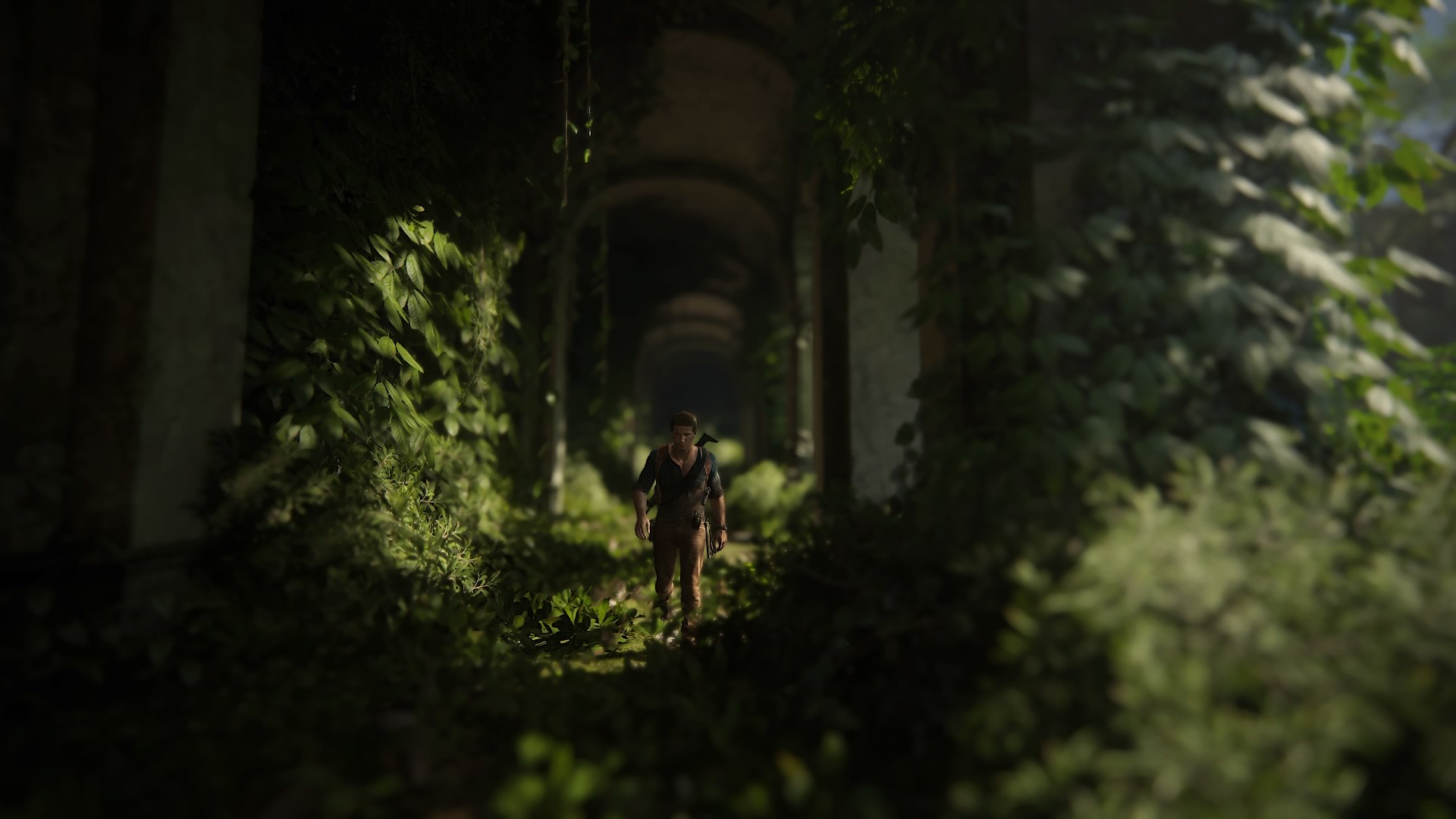The image depicts a highly digitalized, three-dimensional scene reminiscent of a high-definition video game, potentially from the Uncharted series. It features a large, abandoned structure with high ceilings, domed and arched doorways, overgrown with lush greenery, including vines and trees creeping up the walls. Amidst the shadows and soft light playing off the foliage, a man resembling an adventurous explorer — perhaps Nathan Drake — is seen walking down a pathway flanked by concrete pillars. He is notably dressed in brown pants and a t-shirt, with a watch on his wrist and a gun slung over his shoulder, advancing through the undergrowth in what appears to be a mysteriously intriguing temple-like environment.